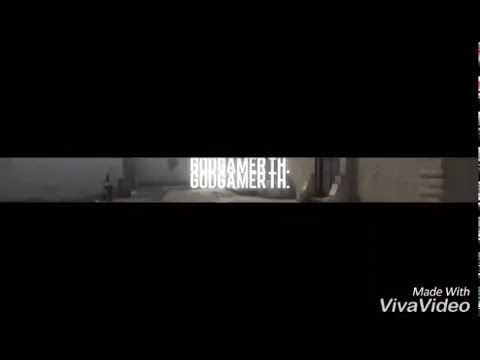The image appears to be a promotional still from a video, possibly one related to gaming or a video game. The overall composition is a rectangle with the top and bottom portions being predominantly black, each occupying about 40% of the total space, creating a shadow effect around the central part of the image. The central section, comprising roughly 20% horizontally through the middle, displays a scene that appears to be a portion of a game map or a battlefield area, predominantly rendered in shades of gray and brown. Across this central section, in bold white capital letters, the text "GOD GAMER TH" is prominently displayed twice, one directly on top of the other. Additionally, in the bottom right-hand corner, there is a watermark that reads "MADE WITH VIVA VIDEO." The background behind the text features elements that resemble a brick or stone structure, possibly depicting an open doorway with concrete borders and a walkway.